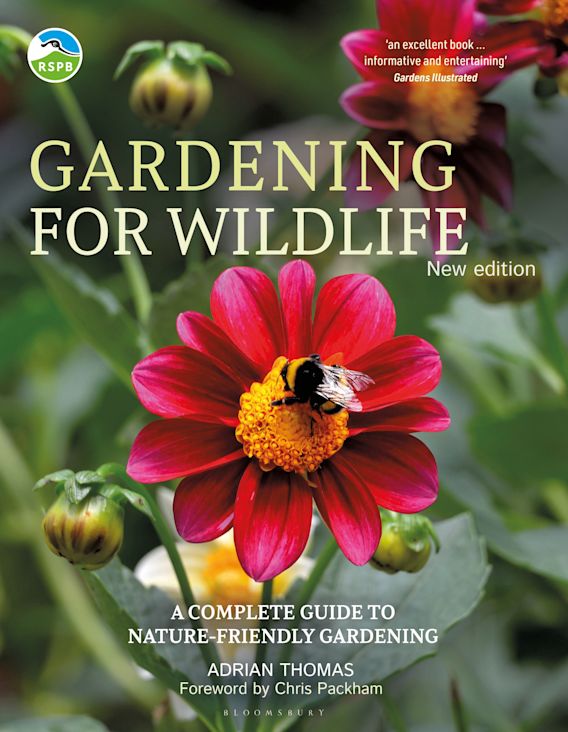The front cover of this rectangular book, measuring approximately 6 inches high by 4 inches wide, features a striking dark pink flower with long petals and a central yellow and white core. A black and yellow bumblebee is perched on the flower’s center. Surrounding the main flower are additional green stems, buds, and petals, with some other pink flowers subtly faded into the background.

At the top of the cover, in a bold white font with a yellow-green shadow, the text reads, "Gardening for Wildlife, New Edition." Directly above this title is an endorsement in smaller print, "An excellent book, informative and entertaining - Gardens Illustrated." On the upper left corner is the logo of the RSPB—a circular emblem featuring a stylized bird with a blue top and green bottom. 

Closer to the bottom of the cover, additional text in white states, "A Complete Guide to Nature-Friendly Gardening," attributed to Adrian Thomas with a foreword by Chris Packham. The book is published by Bloomsbury, as indicated at the very bottom of the cover. This visually rich and informative cover encapsulates the essence of gardening and wildlife, promising an engaging read for nature enthusiasts.